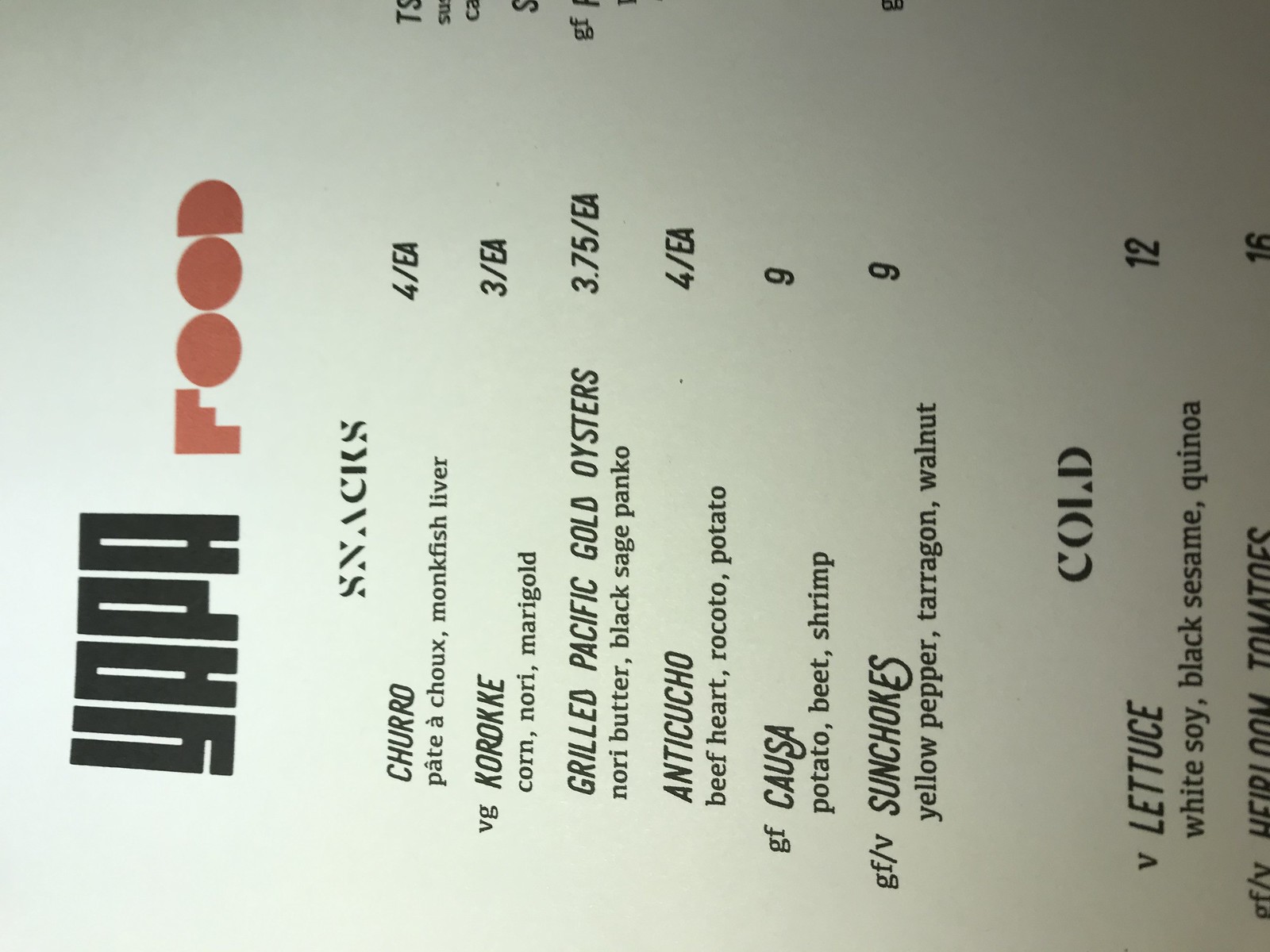The image showcases a visually striking menu from YAPA, presented sideways at a 90-degree tilt to the left. The menu is crafted with an artistic flair, featuring creatively styled fonts in a light brown hue against an off-white background. As you peruse the offerings, the text appears meticulously designed, emphasizing the establishment's unique atmosphere.

The menu is divided into sections, with the top portion dedicated to "Snacks." Among these, items such as "Churro" and "Korokke" (spelled K-O-R-O-K-K-E) are listed, alongside "Grilled Pacific Gold Oysters." The snacks section includes a mix of intriguing and exotic choices like potato, beet, shrimp, beef heart, ricotto, potato, yellow pepper, tarragon, and walnut.

At the bottom, just before the image cuts off, additional items such as "Cold Lettuce with White Soy, Black Sesame, and Quinoa" are visible. The right side of the menu displays numbers indicating quantity and price (e.g., four per each, three per each, 3.75 per each, nine, and twelve), although some menu items in this section are partially cut off by the image's frame.